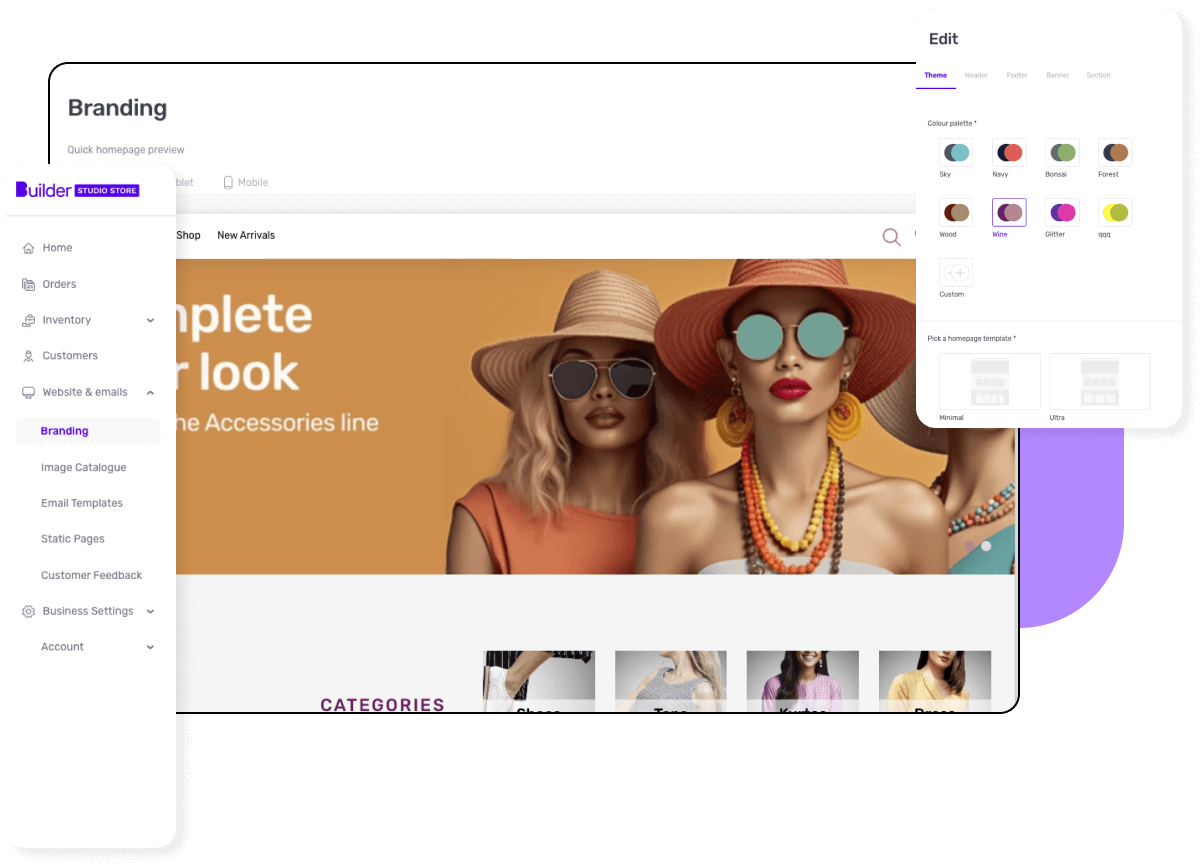A vibrant webpage dedicated to fashion, prominently displaying a variety of colorful offerings. The upper left corner of the interface features a navigation panel including options such as branding, quick home page preview, builder, home orders, inventory, customizers, website and emails, branding, image catalog, email templates, static pages, customer feedback, business settings, and account management. A highlighted menu item reads "Complete Your Look: The Accessories Line", suggesting active selection. The central image showcases three women donned in large hats and mirrored sunglasses, exuding sophistication and mystery as their eyes remain concealed. Each woman wears outfits in distinct colors, emphasizing the website's emphasis on vibrant fashion choices. On the upper right corner, there are tools for editing and a palette of color swatches for customization. Directly beneath the image, categories are neatly listed, possibly including shoes, tops, sweaters, and blouses, providing easy navigation for the user.